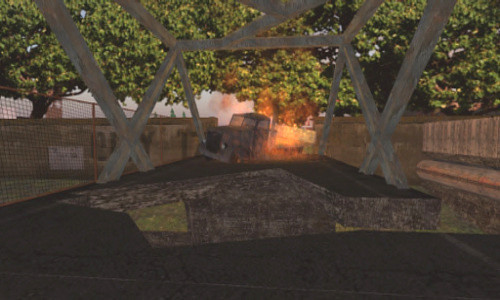The image is a low-quality, computer-generated scene reminiscent of a video game or cartoon. In the background, a number of big green trees stand tall, creating a natural setting. Ahead of them, a brown wooden or chain-link fence stretches across the image from left to right. At the very center of the image, an old, grey, 50s-style pickup truck with a black grill is caught in a fiery blaze at its back end, emitting orange flames. The foreground features a broken, dark grey asphalt surface, with patches of lighter grey and a small area of green grass to the left. Adding a geometric complexity, light-colored X-shaped beams extend upwards to form a square-like structure. The entire scene, devoid of people, suggests a dramatic moment captured in broad daylight.